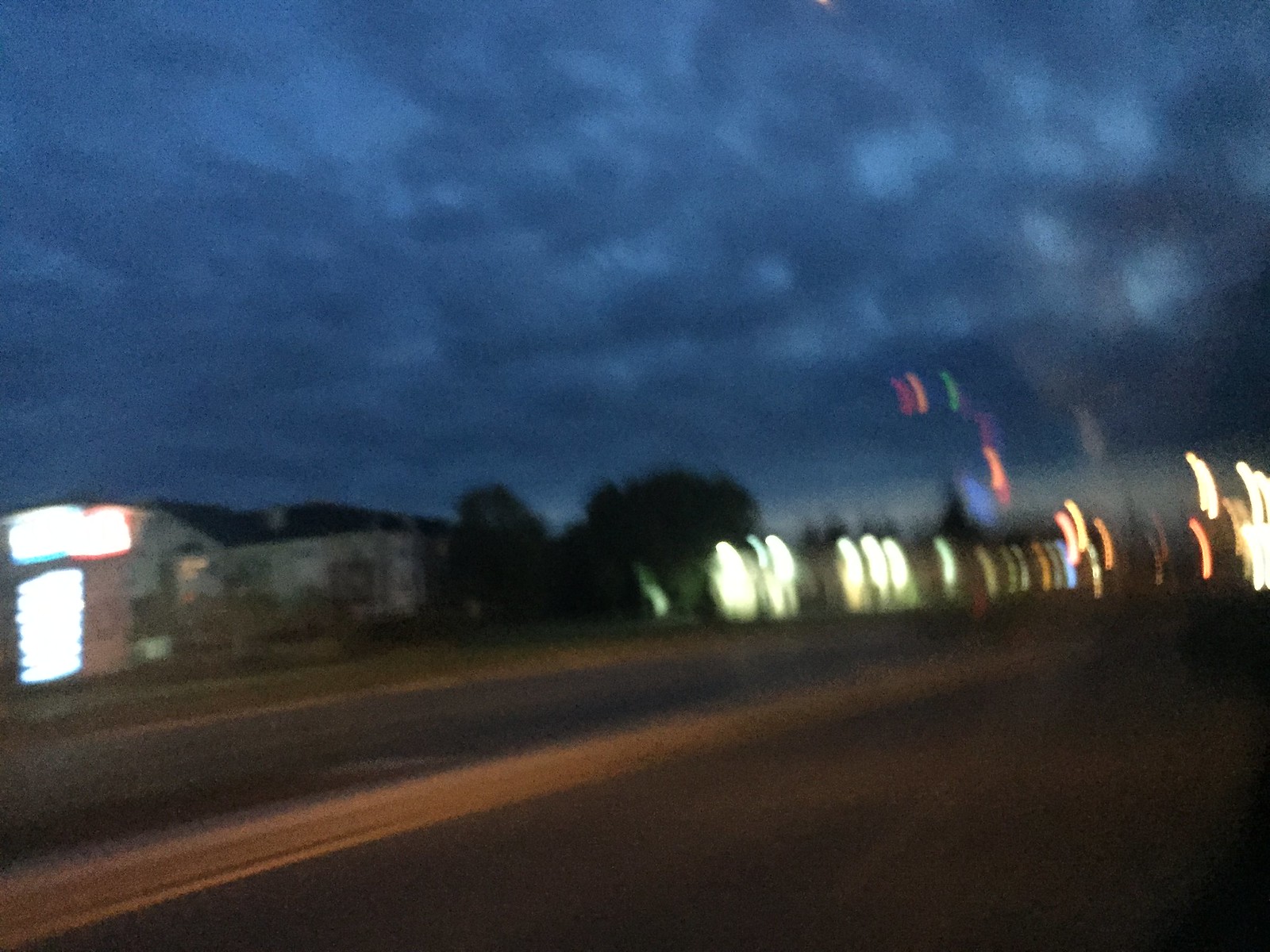This blurry nighttime outdoor photograph captures a scene that is difficult to discern clearly. At the top of the image, a dark blue sky transitions towards a bluish-black hue suggestive of either dusk or dawn, filled with clouds that obscure any stars or the moon. Below the sky, a row of trees stretches across the image, partially obscuring a building. The building has a light in front of it, further illuminating its surroundings. In front of this building and the trees lies a highway adorned with various lights. 

To the right, the highway lights appear to scatter in different colors, including white, red, orange, blue, and purple. These may be from oncoming traffic or other light sources, contributing to the blurry, motion-filled look of the photo. More towards the left of the highway, a blue-roofed, two-story hotel with white brick can be seen. It has an illuminated sign out front, though the text is too blurry to read. Beside the hotel, there are additional red and blue lights, likely from a sign. The photograph overall depicts a scene filled with various indistinct lights and structures, contributing to its enigmatic and obscure quality.